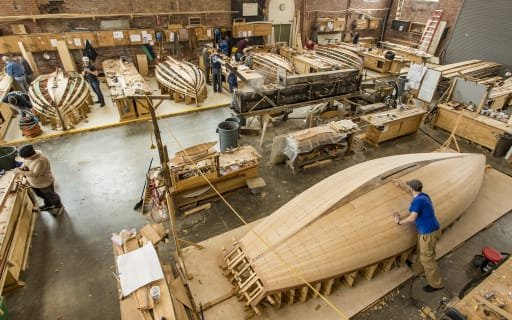The image depicts a bustling woodworking shop focused on boat manufacturing, showcasing an environment filled with the light brown hues of the wood and the slightly darker tones of the stone floor. Prominently in the foreground, a man wearing khaki pants and a blue shirt appears to be sanding the bottom portion of an upside-down, small wooden boat, which features a dark brown strip of lining through its center. This main worker is joined by another man in a white shirt on the left, and both are part of a larger group of men, all dressed in casual work attire with hats, t-shirts, khakis, or jeans, actively engaged in various stages of boat construction. The shop is devoid of large machinery, instead brimming with handheld tools, numerous wooden stands, and cubbies in the background filled with wood planks and other materials. A yellow string-like object stretches from the center to the bottom right portion of the image, and a small part of a gray wall is visible to the right. The image captures the intricate, hands-on craftsmanship involved in creating these wooden boats.